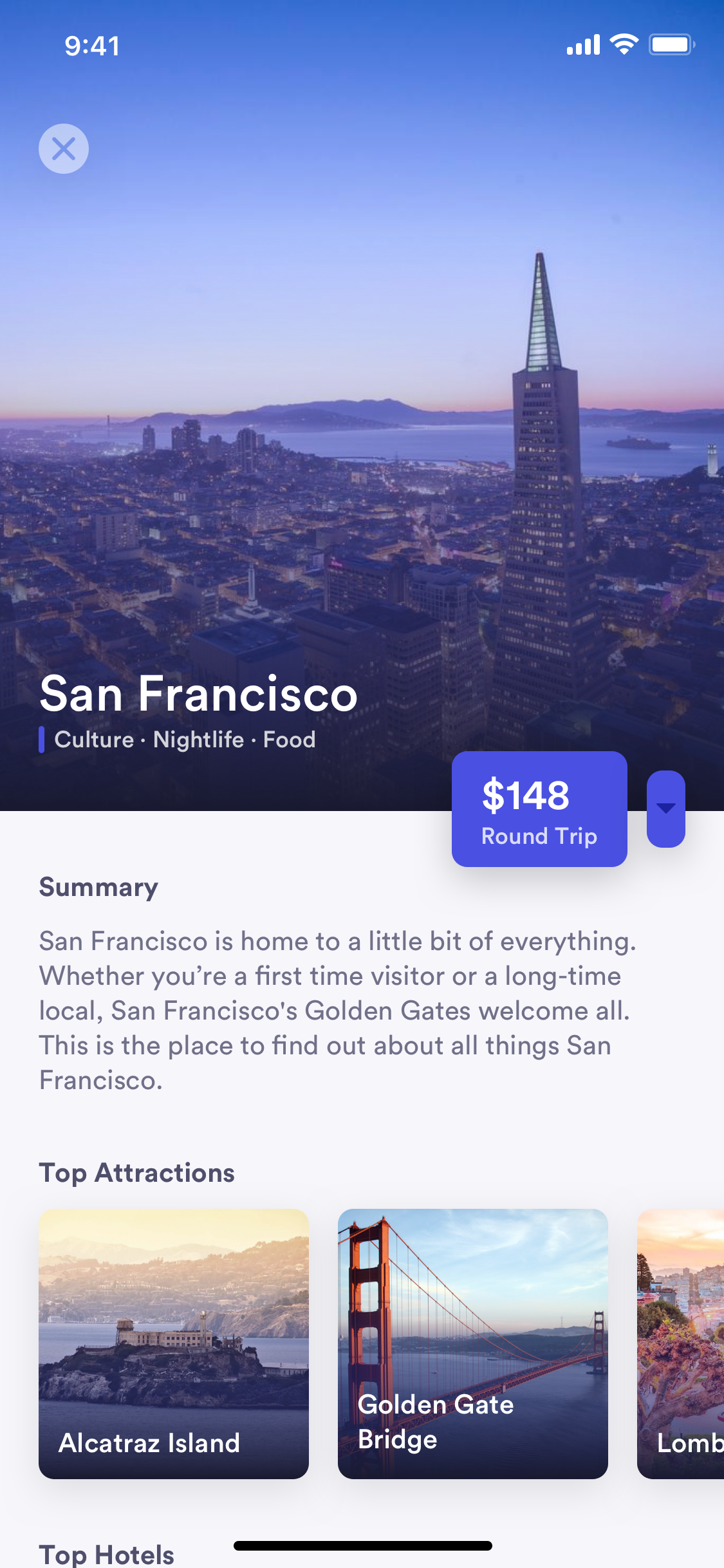The screenshot captured from a phone displays various elements and information related to San Francisco. The top left corner shows the time as 9:41. Below the time, there is a striking image of the San Francisco skyline viewed from across the bay, with distant mountains and either a sunset or sunrise illuminating the scene. The screenshot prominently features text which reads, "San Francisco Kosher Nightlife Food $148 for a round-trip."

Directly beneath this, a white box contains the summary: "San Francisco is home to a little bit of everything, whether you're a first-time visitor or a longtime local. San Francisco Golden Gate welcomes all. This is the place to find out about all things San Francisco." 

Further down, the screenshot highlights various attractions with "Top Attractions" heading a section. A square box showcases an image of Alcatraz Island, and to its right, an image of the Golden Gate Bridge against a clear blue sky. 

Below this, on the left side, the heading "Top Hotels" is visible, accompanied by a black stripe running horizontally across the screen.